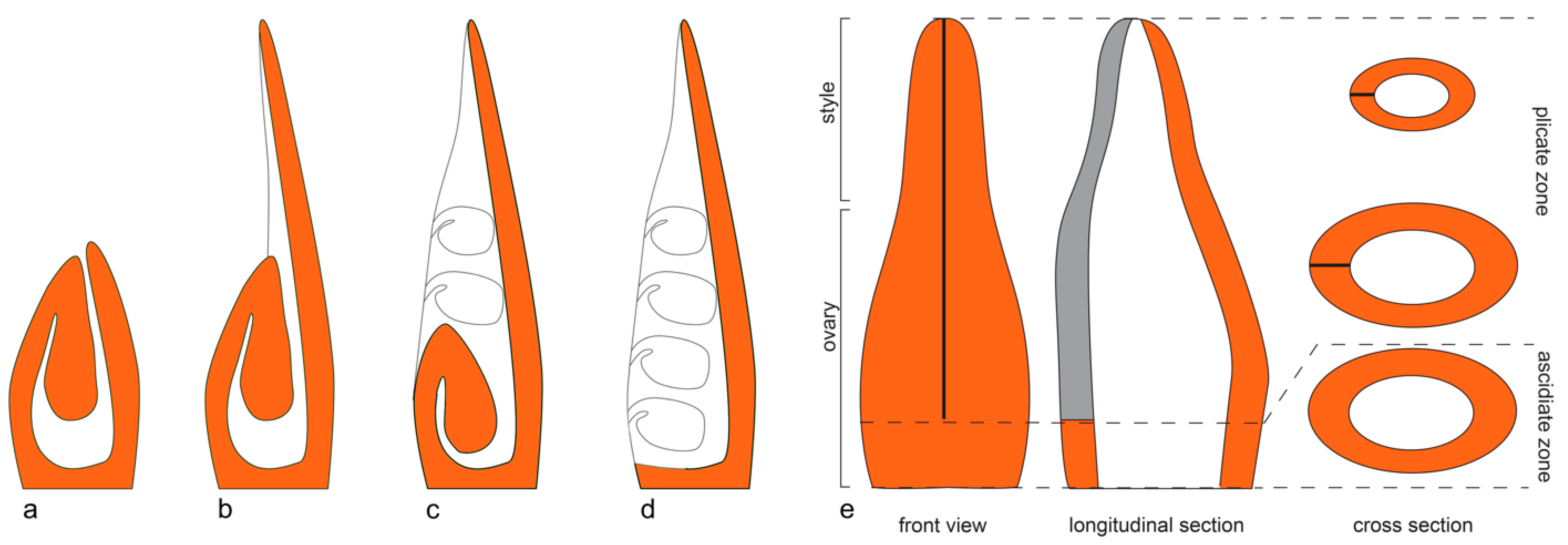The image showcases a detailed scientific diagram of the developmental stages of what is likely a peapod plant. The illustration is presented with a white background and features figures A through E, depicting the growth process in vibrant orange and thin black lines. 

- **Figure A**: This is a depiction of the plant in its initial stage, showing a closed bud with a distinct white swirl in the middle.
- **Figure B**: The bud on one side has grown long and extends upward to the top of the picture.
- **Figure C**: The plant now reveals thin lines reaching down with two white swirly features inside, indicating the development of seeds or pods.
- **Figure D**: At this stage, the plant is fully extended, showcasing four white pods in the middle.
- **Figure E**: This figure provides detailed annotations for parts of the plant, including the ovary, style, front view, longitudinal section, cross-section, pillicate zone, and acid dilate zone.

Additional diagrams on the right side of the image display three horizontal, oval-shaped objects highlighting specific botanical features, further elaborated by vertical texts labeling key zones and sections of the plant. The comprehensive labeling across the figures provides a thorough understanding of the peapod plant's growth from bud to fully developed pods.